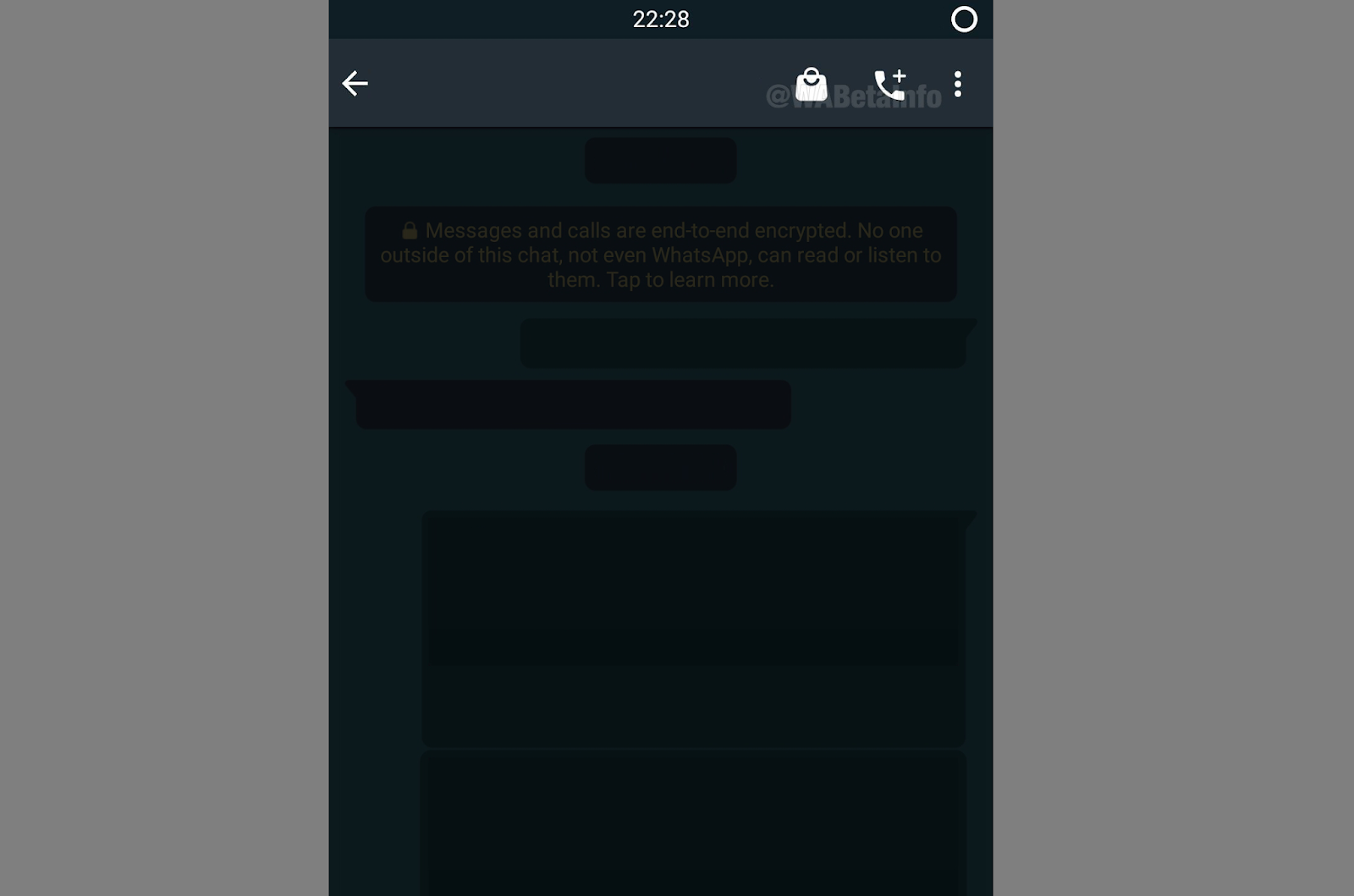This image is a screenshot taken from a mobile phone, displayed against a medium gray, landscape-oriented rectangular background. The central screenshot has a predominant bluish tint. At the top of the screenshot, there is a black header displaying the time "22:28" in white text centered in the middle. In the top right corner, there is a white circular outline icon.

Below the black header, a lighter bluish gray header hosts additional icons. On the left side, there is a white arrow pointing to the left. On the right side, there are three icons: a white shopping bag icon, a white phone icon with a plus sign angled upwards to the right, and three vertically stacked white dots.

Superimposed over this header, a watermark reads "@WA.beta.info" in very light, translucent white text.

The main body of the screenshot features a very dark bluish background. At the top center, there is a small, black rectangle with rounded corners. Below it, a larger black rectangle with rounded corners contains dark gold text and a dark gold lock icon. The text is spread across three lines and reads: "Messages and calls are end-to-end encrypted. No one outside of this chat, not even WhatsApp, can read or listen to them. Tap to learn more."

In the conversation area beneath this notice, there is a green speech bubble icon with its pointed part extending from the right side of the frame, indicating outgoing messages. This pattern continues throughout the conversation thread.